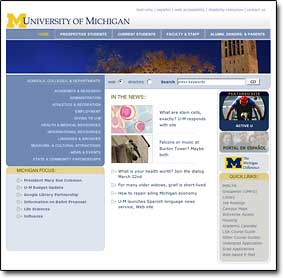This image depicts a zoomed-out view of the University of Michigan homepage. In the top left corner, an iconic yellow "M" logo is prominently displayed next to the phrase "University of Michigan" in blue text. Beneath this header, there are five categories arranged horizontally, with the leftmost category highlighted in yellow while the remaining four are white. 

The main section of the webpage features a dark blue background adorned with the upper portion of a tree and a tower, which provides a picturesque backdrop. To the left of this section, a blue square contains what appears to be ten white sub-categories, each with its own descriptive text. Below this, another square in gray offers additional navigational options.

At the center of the page, a white backdrop showcases two clickable links, each accompanied by an image on their left side, indicating their interactive nature. Above these links, the section is labeled "In the News," and directly below are four additional links, likely leading to various articles or web pages.

Above this main content area, a search bar is prominently featured with a silver "Go" button beside it, facilitating easy navigation. On the right side of the image, another Michigan logo is present, followed by a yellow headline. Below, a set of smaller categories appear against a gray background, situated in the bottom right corner of the screen.